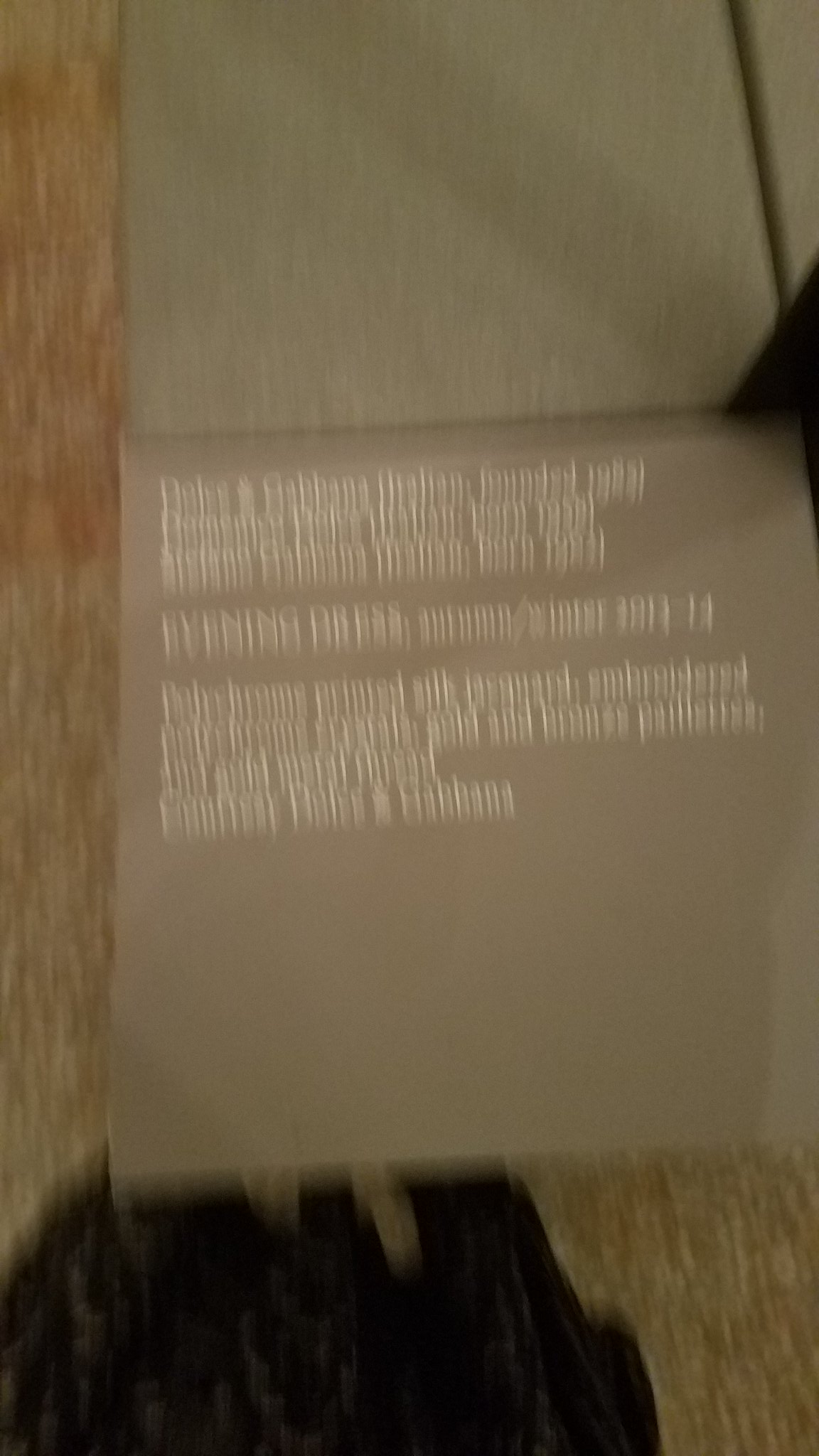This image is a poorly taken, blurry photo that seems to capture a museum exhibit or display in motion. The main subject appears to be a sign or a piece of text showcasing information about Dolce & Gabbana, specifically mentioning "Italian founded 1980" and possibly "evening dress." The sign is situated near a bench area. Below the sign, on a tannish-white floor, there is a noticeable black plastic bag. The photo also includes indistinct gray tiles or squares that are separated by some sort of metal divider. The blur and low quality of the image make the text largely unreadable and suggest it was taken while the camera was moving.